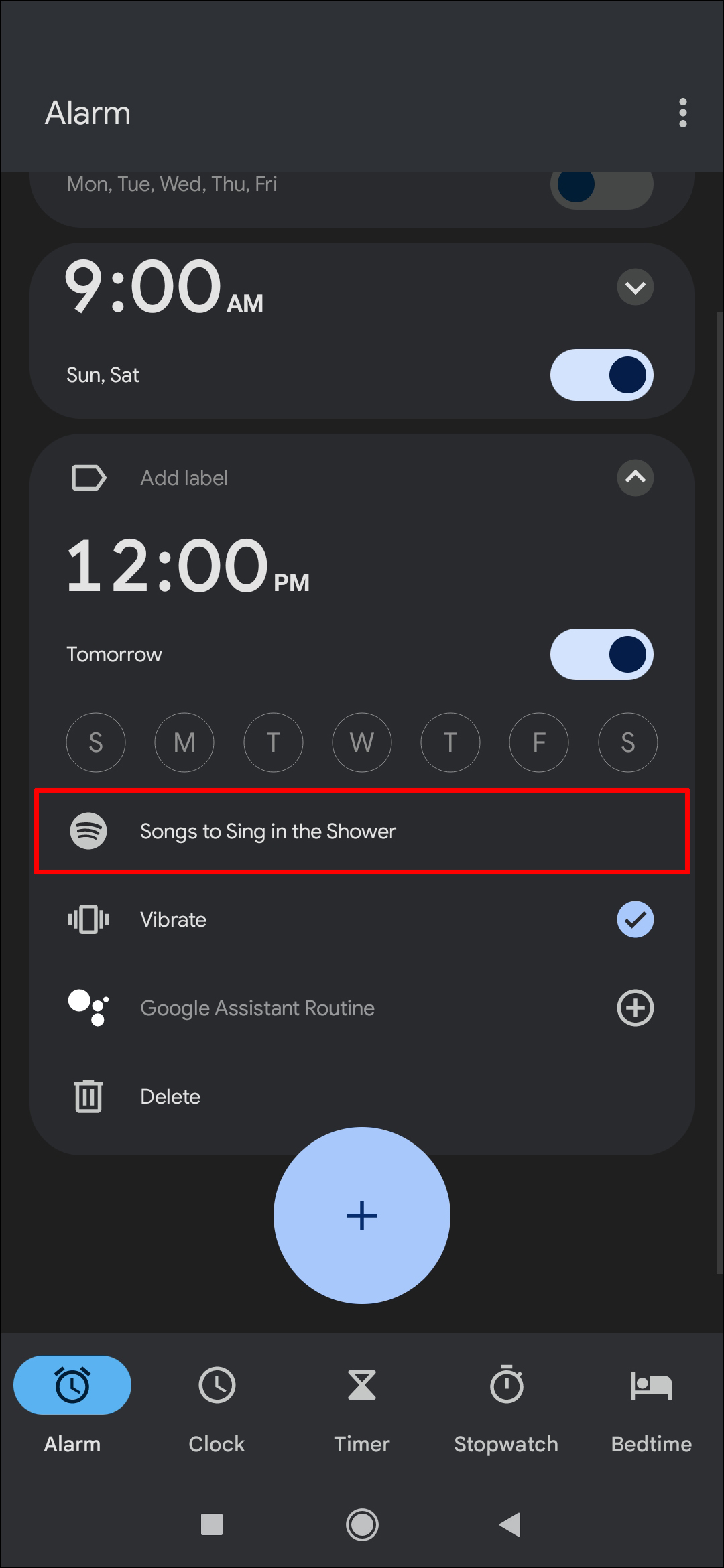The phone screen displays the alarm settings. The screen shows alarms set for Monday, Tuesday, Wednesday, and Friday, with a start time of 9:00 a.m. for both Saturday and Sunday. An option to "Add Label" is visible, with a note for "12 p.m. tomorrow" highlighted. There's a red box around an item labeled "Songs to Sing in the Shower," indicating it's an alarm label or playlist. The "Vibrate" option is checked off, and the "Google Assistant Routine" setting is visible below that. At the bottom of the screen, there is a "Delete" option. A blue circle with a plus sign inside is underneath this section, indicating the option to add a new alarm. On the bottom row of the screen, there's a blue bar featuring an alarm clock icon, alongside other icons: a white clock, a white timer resembling an hourglass, a stopwatch, and a bedtime mode symbol with a bed and a person in it.